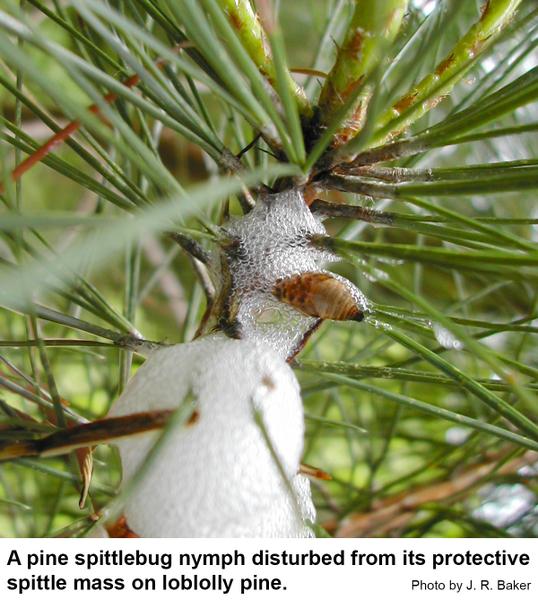The image captures the detailed scene of a loblolly pine tree with its vibrant, well-maintained branches spreading out in various directions. The captivating green hues of the pine's needles range from light to dark, creating a harmonious blend of colors that stand out distinctly. At the center of the composition is a pine spittle bug nymph, which appears to be in distress after being disturbed from its protective spittle mass. The nymph is enveloped in a frothy, rich foam that serves as its defensive habitat. The spittle-bug nymph's presence adds a touch of intrigue and biological interest amidst the lush, prickly leaves of the pine tree.